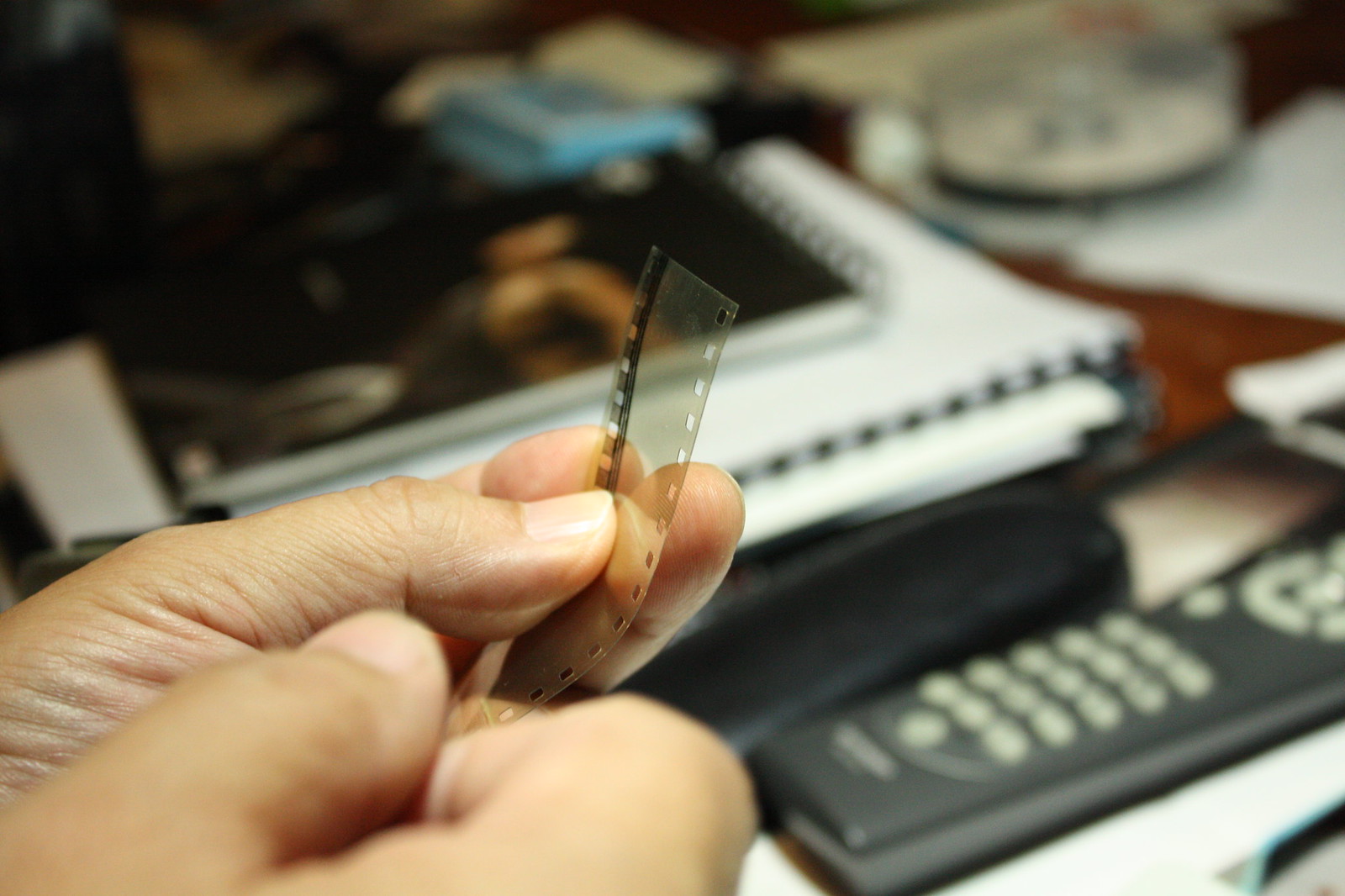In this detailed color photograph, a man's hands are prominently featured in the bottom left corner. His left hand is holding a clear, grayish film strip pinched between the thumb and middle finger. The film strip has distinctive black edges and notches on both sides, reminiscent of old camera or microfilm film that requires development. The background, which is blurred to keep the focus on the hands and the film, reveals a cluttered tabletop surface, presumably a wooden desk, scattered with various objects. Among these, a black television remote is clearly visible in the bottom right corner. Behind the hands, there's a hint of stacked books with white and black trim, along with other indiscernible items, all contributing to the photographic style of representational realism. The lighting in the image highlights the intricate details of the film and the texture of the man's hands, creating a sense of intimacy and focus on the act of examining the film strip.